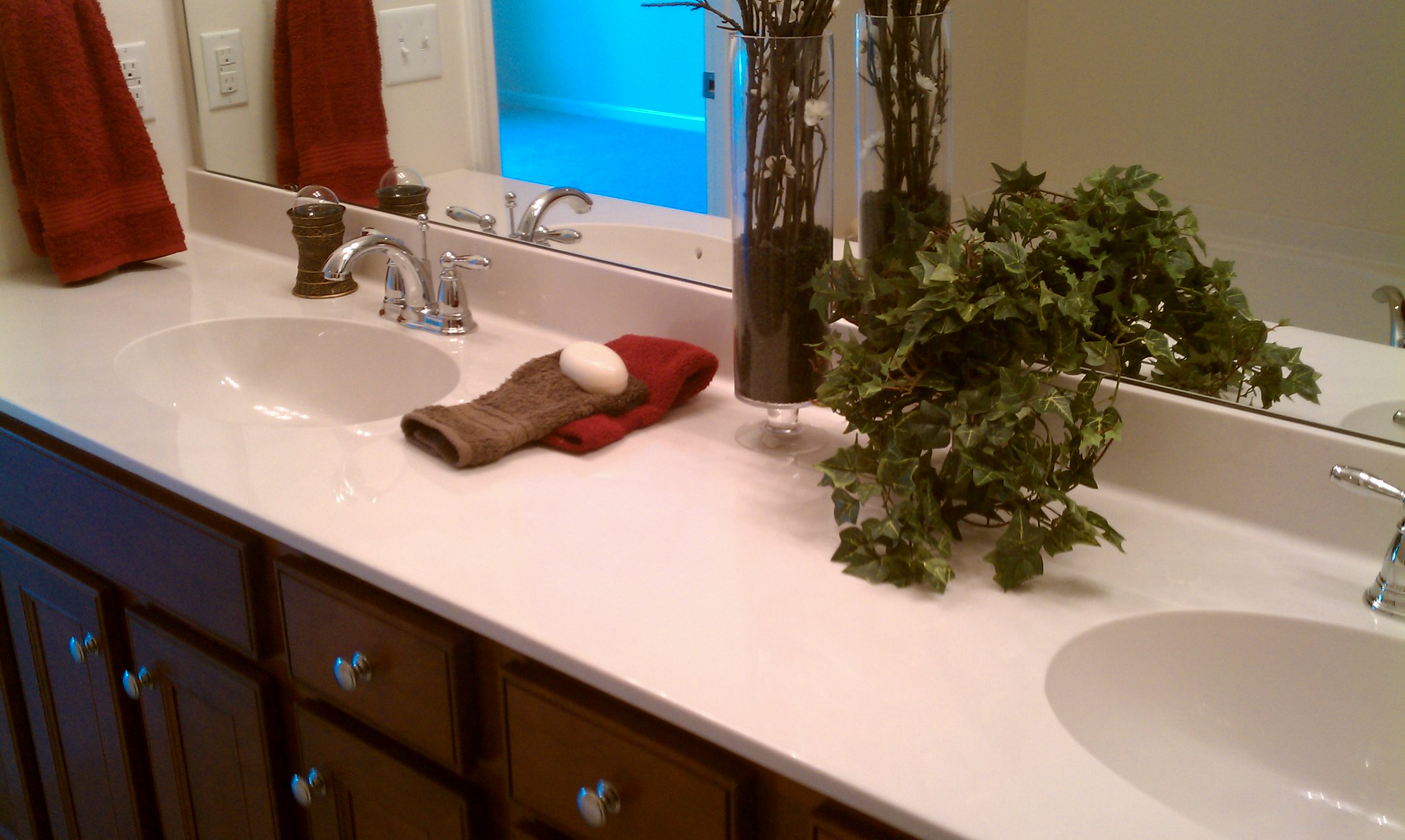The digital photo captures an indoor bathroom scene with meticulous detail. On the right side of the image, there's a large mirror reflecting part of the room. In the upper left corner, a neatly hung brown hand towel stands out against the cream-colored wall. Below the towel and to its right, a white electrical outlet is visible. The countertop starts on the left side of the photo, extending across until it dips down to accommodate a white sink. The sink itself features a silver faucet with two coordinating handles. 

To the left side of the sink, another brown hand towel lays flat, serving as a resting spot for a white bar of soap. Adjacent to this, a clear pedestal holds a dark brown vase—seemingly filled with dirt—topped with a green ornamental plant. Another leafy green plant is positioned to the right of this setup, adding a touch of nature to the scene. 

In the bottom left corner, dark brown cabinetry is visible, featuring several drawers and two cabinet doors, all outfitted with functional silver handles. Six silver knobs, also for opening the drawers and cabinets, are neatly aligned. Reflecting in the mirror near the hand towel, a dual light switch is visible, showing one switch in the 'on' position and the other 'off'. The mirror also captures the partial reflection of a white door that opens into a neighboring bedroom, distinguished by its blue carpet and strikingly bright blue walls.